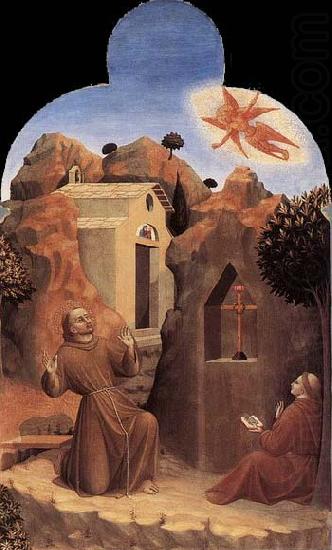This vertical, rectangular painting vividly portrays a sacred scene with two monks positioned in prayerful postures against a backdrop of brown stone formations, lush trees, and a distant city that includes structures like a chapel or a monastery. The monk on the left is kneeling, hands raised in reverence, gazing towards an ethereal angel that soars overhead, encircled by a radiant golden glow against a blue and white sky. This angel, distinguishable by its wings, exudes a spiritual presence. The monk on the right, identifiable by his tonsured (shaved) head with a ring of hair, sits contemplatively against a tree, a book in hand, with one palm extended upwards. Both monks wear traditional brown robes cinched at the waist. Central to the scene is a carved stone alcove holding a simple, brown crucifix. The absence of text on the image allows the rich hues of tan, brown, blue, white, black, gold, and off-white to convey the solemn and reflective atmosphere of this religious tableau.